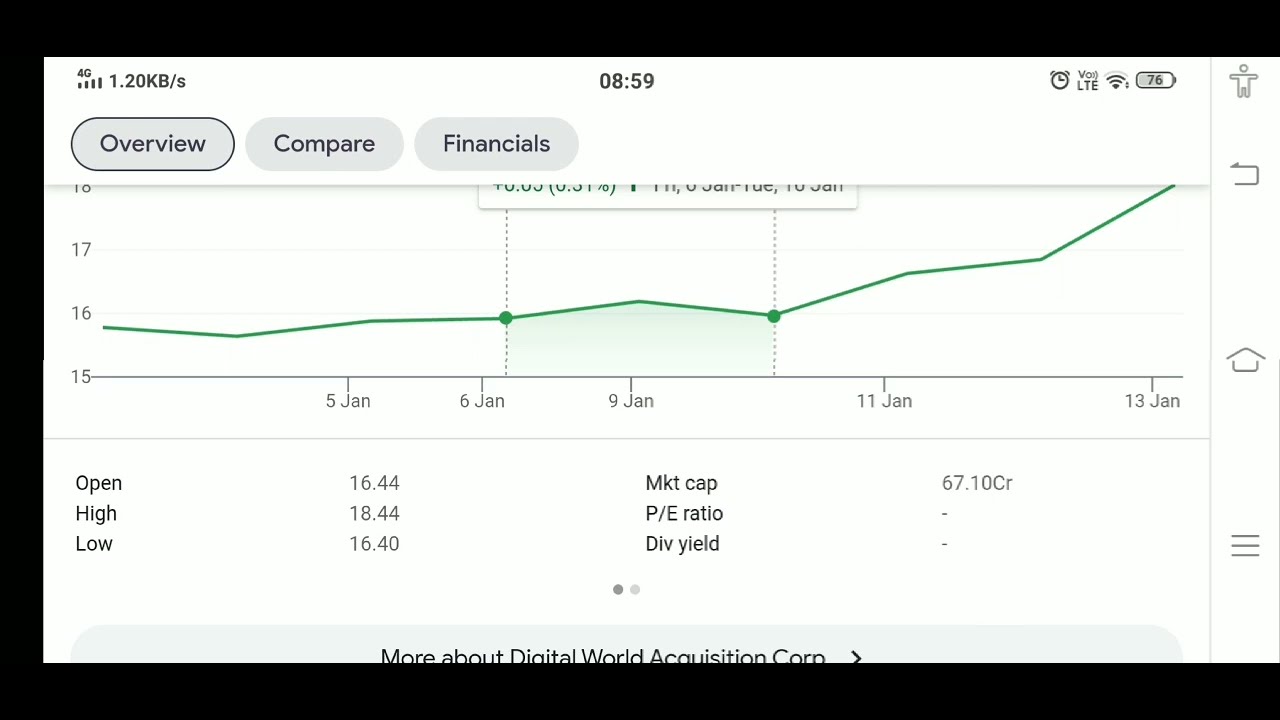The image depicts a screenshot of a computer application, framed by black borders on the top, left, and bottom, with a white sidebar on the right containing various icons including a small clock, "LTE", Wi-Fi strength meter, and a battery indicator at 76%. At the top left of the screen, the number 40 is displayed alongside a meter that ranges from small to larger ticks, showing a rate of 1.20 kb/s. Centrally positioned at the top is the time stamp "08:59". Below this, in gray ovals, are the options "Overview," "Compare," and "Financials".

The main feature of the screenshot is a line graph. On the vertical axis, the numbers range from 15 to just visible 18, increasing by ones, while the horizontal axis is marked by dates: 5 Jan, 6 Jan, 9 Jan, 11 Jan, and 13 Jan. The green line of the graph, annotated with green dots on specific points (6 Jan and around 10 Jan), moves from just below 16 and ascends towards January 13th. Light blue shading is present underneath the line between these green dots, emphasizing the graphical data.

Beneath the chart, a section lists the values "Open 1644," "High 1844," and "Low 1640." Further right, additional financial metrics are provided: "MKT cap" at 67.10 CR, "PE ratio," and "Dividend yield," though the latter two values are not fully visible. The bottom of the image shows the text "More about Digital World Acquisition Corp," in a purplish hue, partly obscured by the border.